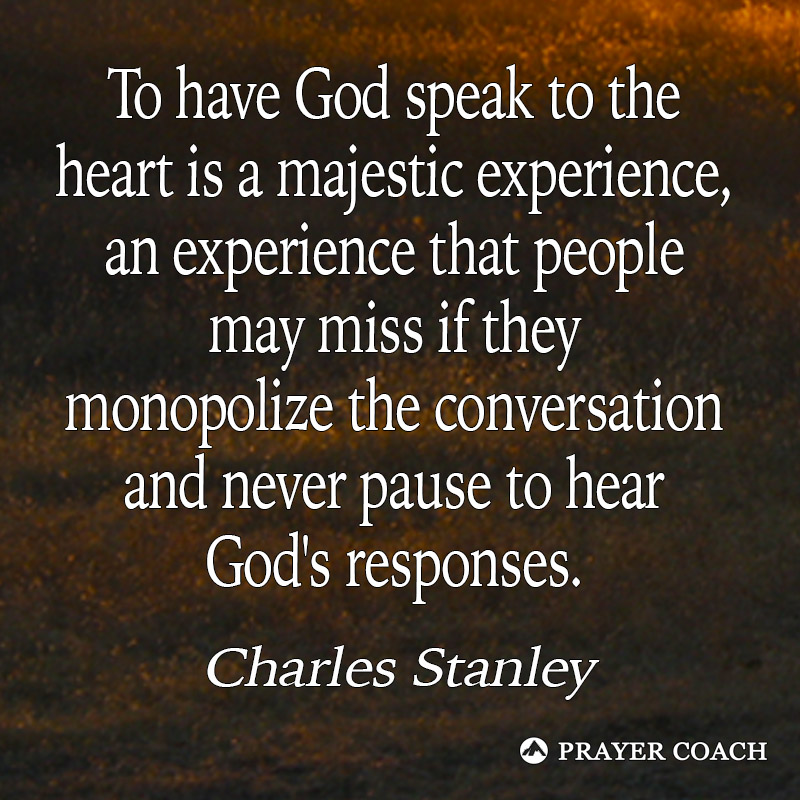The image features a digitally created gradient background with varying shades of brown, giving it a striped appearance as the light and dark browns fade into each other. Overlaying this background is a prominent quote in white text that reads, "To have God speak to the heart is a majestic experience, an experience that people may miss if they monopolize the conversation and never pause to hear God's responses." This quote is attributed to Charles Stanley. Below the quote, in the bottom right corner, more white text reads, "prayer coach." To the left of this text is a circular white logo featuring the silhouette of a mountain. The image has a slightly grainy or foamy texture, adding depth to the background. The photograph appears to be a digital marketing piece, possibly a social media post, captured in a way that focuses directly on the text, with all elements centered for emphasis.